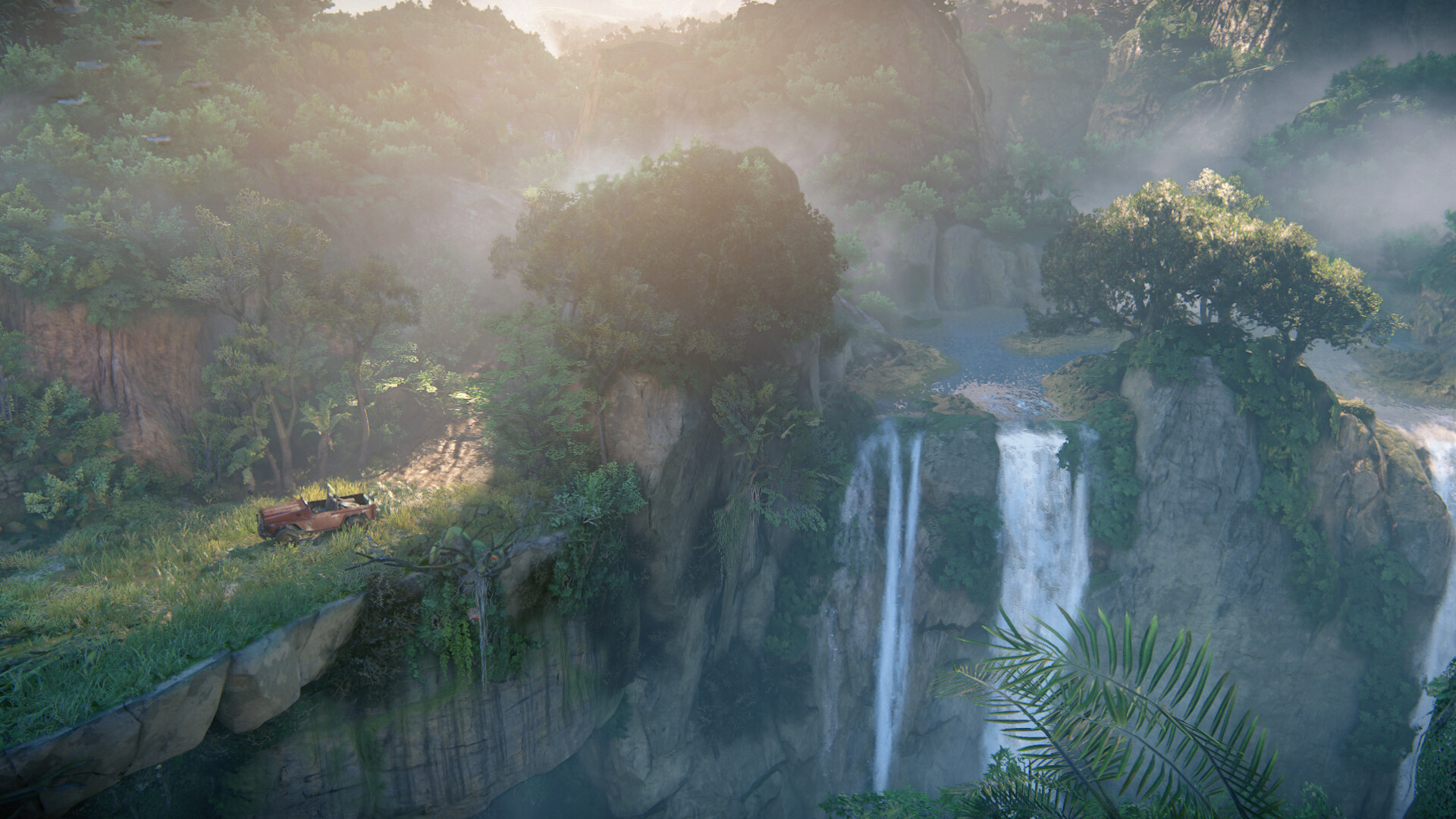"Digital Rendering of a Mystical Rocky Cliffside with Waterfalls and Foliage: 

This stunning digital artwork, potentially concept art for a video game or a movie, showcases a meticulously detailed rocky cliff face adorned with lush leaves and vines cascading down its rugged sides. Two majestic waterfalls dramatically spill over the cliff edges—one centrally positioned and the other towards the far right—each contributing to the ethereal, misty haze that envelops the surrounding greenery. In the foreground, an orange Jeep-like vehicle rests in a grassy area to the left, adding a pop of color and a sense of scale to the scene. The image captures a serene yet adventurous atmosphere, inviting the viewer into this vividly imagined natural landscape."